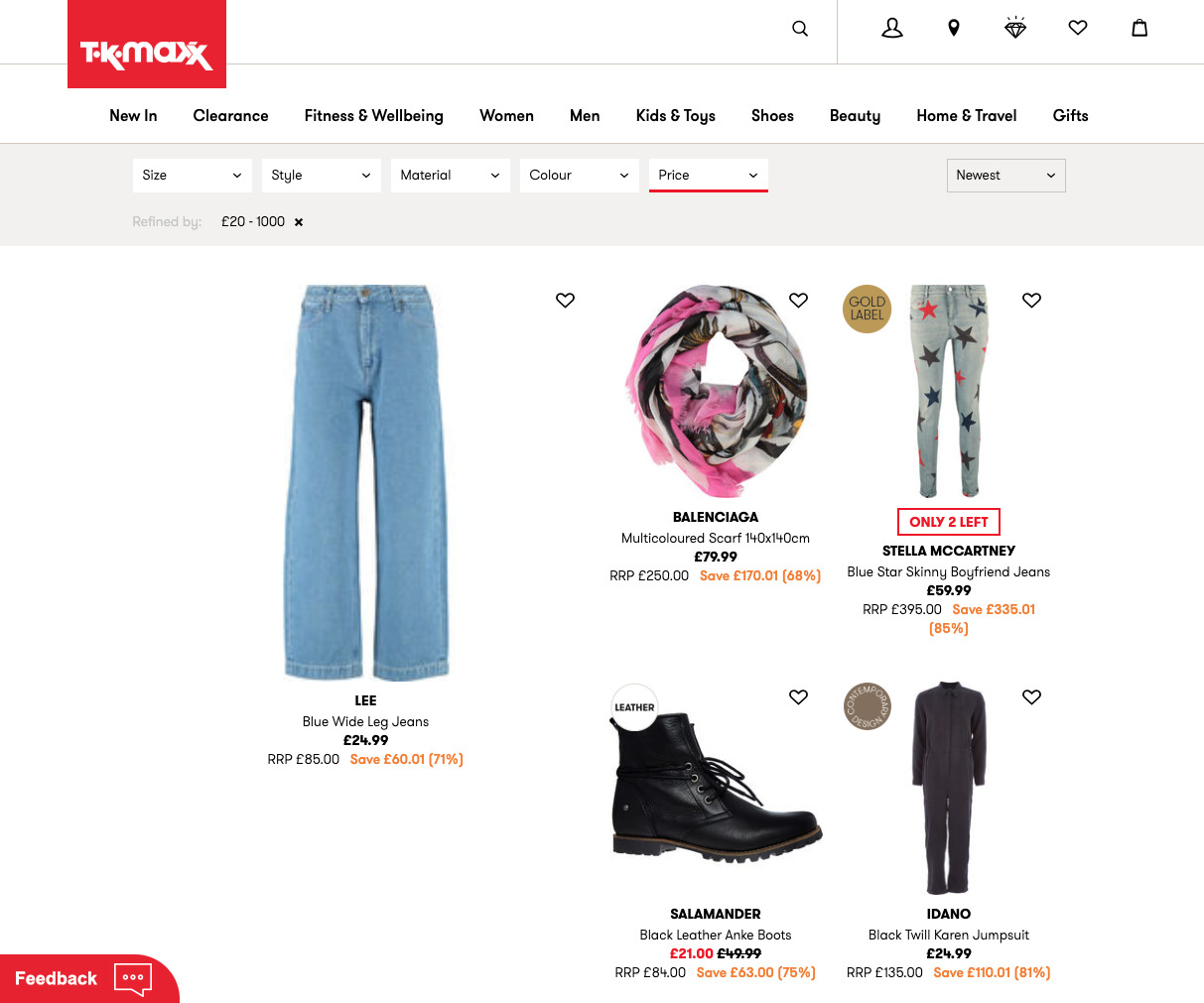In this image, we see the storefront of TK Maxx. Positioned at the top left corner of the image, the store's name, "TK Maxx," is displayed in bold white letters against a vivid red background. Just below this header, extending from left to right, are the store's different categories: "View In," "Clearance," "Fitness and Well-being," "Women," "Men," "Kids and Toys," "Shoes," "Beauty," "Home," "Travel," and "Gifts."

Beneath these categories, there's a large rectangular section spanning the width of the image. Inside this section are several filters to assist with shopping, labeled from left to right: "Size," "Style," "Material," "Color," and "Price"—with the "Price" filter underscored by a red line.

Moving to the bottom middle portion of the image, we see a display of products available in the store. On the far left are blue jeans labeled "Wide Leg Jeans," priced at $24.99. To the right of the jeans are four more clothing items, each distinctly pictured, and placed next to a singular boot on the bottom left of this grouping. The scene captures a detailed snapshot of the store's online interface, showcasing both product categories and specific items available for purchase.